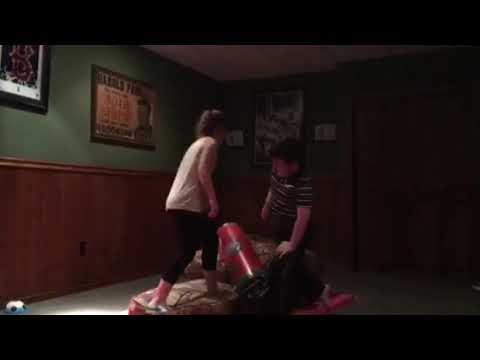This picture depicts an indoor setting with wooden panels on the lower part of the wall and a green section above, adorned with posters and photographs, likely showcasing sports figures. In the center of the image, there are two individuals—a woman on the left and a younger boy on the right—in a somewhat chaotic setting. The woman, dressed in a light t-shirt and dark pants, appears to be walking atop various indistinguishable objects scattered on the floor. The boy, wearing a striped dark shirt and black pants, is crouched down, with his left arm resting on his knee, oriented towards the woman. Between them lies a large, cylindrical, orange-and-green object that looks somewhat like a pop can but might be a trash can or some other type of container. The overall image quality is low, being blurry and grainy, adding to the difficulty in clearly identifying the objects strewn around. On the bottom left corner of the image, a soccer ball is partially visible. The dim lighting further complicates clarity, creating a somewhat mysterious atmosphere in this presumably old photograph.